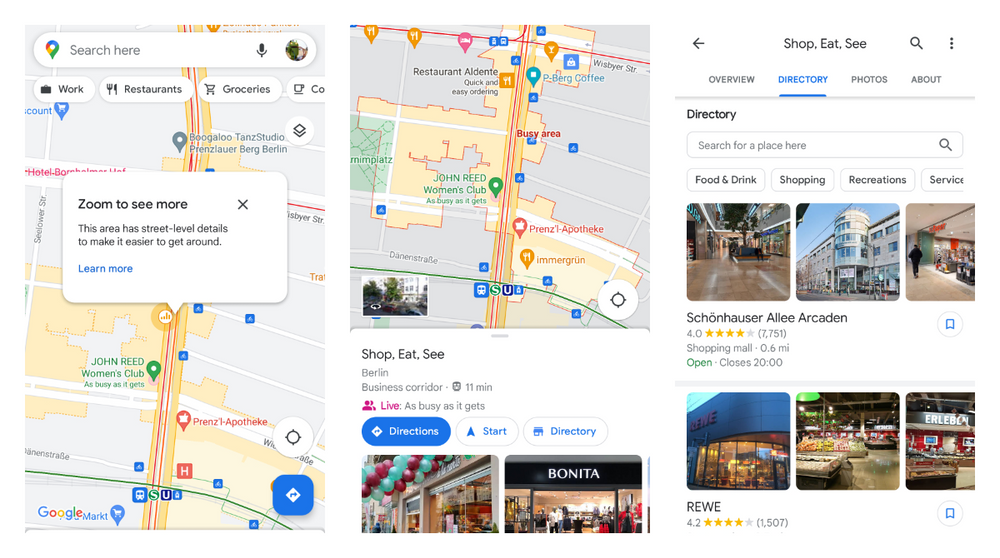This series of three detailed screenshots presents various features of Google Maps in color. 

### Left Screenshot:
The leftmost image highlights a typical Google Maps interface. At the top is an empty search bar, ready for user input. Below the search bar, a detailed map displays several locations: John Reed's Women's Club, a hospital, Boogaloo Tan Studio, and Berg Berlin. A prominent white rectangular pop-up, containing black text, overlays the map and reads, "Zoom in to see more. This area has street-level details to make it easier to get around."

### Middle Screenshot:
The central image also illustrates the Google Maps interface, but with a focus on a particular location. The area under the search bar identifies itself as "shop CE" and "Berlin Business Corridor." The interface includes buttons labeled "Direction," "Start," and "Directory." Accompanying text and images underneath these buttons showcase two different shops.

### Right Screenshot:
The rightmost screenshot shifts to a more specific directory view within Google Maps. The interface, which has a white background, mentions "shop CE" at the top. Tabs labeled "Overview," "Directory," "Photos," and "About" are visible, with the directory tab currently active. This section includes a search bar followed by buttons for specific categories like "Food," "Shopping," "Recreation," and "Services." The screen displays six photographs in two rows of three each, with the second row's images labeled "REWE."

Together, these screenshots provide a comprehensive look at various functionalities within Google Maps, from general navigation and location details to specific shop information and directory listings.